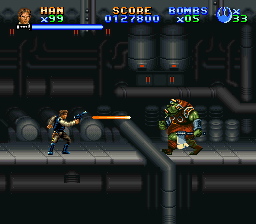This is a detailed animated screenshot from a video game, reminiscent of an arcade style. The backdrop features an industrial setting with complex piping and a platform. 

At the very top of the screen, there's a lit-up statistics bar. On the left side, there's a prominently displayed picture of a man with brown hair and white skin. His name, "Han X 99," is lit up in vibrant orange and yellow text, reminiscent of Han Solo from Star Wars. To the right of his name is a green "99," highlighting his status or level. His icon is adjacent to a blue progress bar illuminated in blue. 

Directly below this interface, the current score is visible, marked in yellow and reading "0127800." There’s also a notation for bombs available, indicating "x 05."

In the scene, Han, dressed in camouflage attire, is positioned on the far left of the screen, facing right. He is engaged in combat, shooting an orange bullet at a large adversary. The enemy, positioned further right across the platform, is a green monster clad in red clothing and wielding an axe. The bullet is captured in mid-flight, adding a dynamic action element to the image.